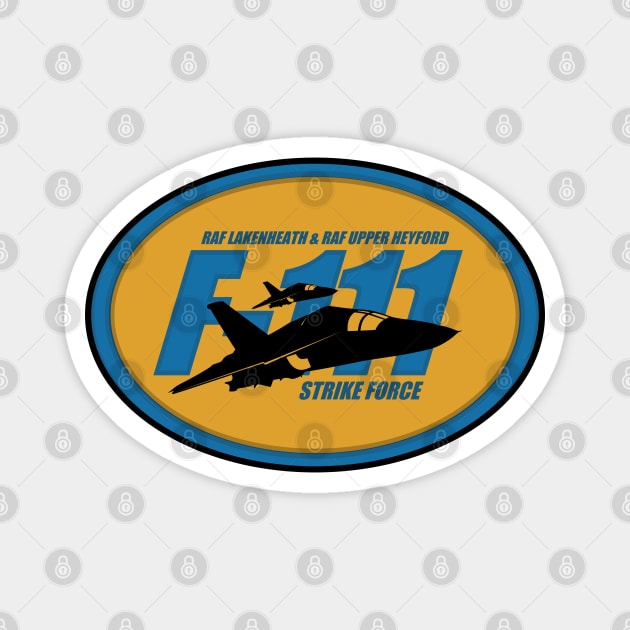The image showcases an oval sticker, which appears to be a product image with a padlock watermark overlay for anti-theft. The sticker has a white border, followed by a thin black line, and then a thicker blue line. The central part of the sticker is gold. Two black jet silhouettes fly across the middle, one appearing larger and closer, and the other smaller and further away. Both planes have geometric, square-shaped fronts and visible yellow windshields. Surrounding the jets, blue text reads "RAF Lakenheath" and "RAF Upper Heyford" above, and "F-111 Strike Force" below. The background of the image is white.